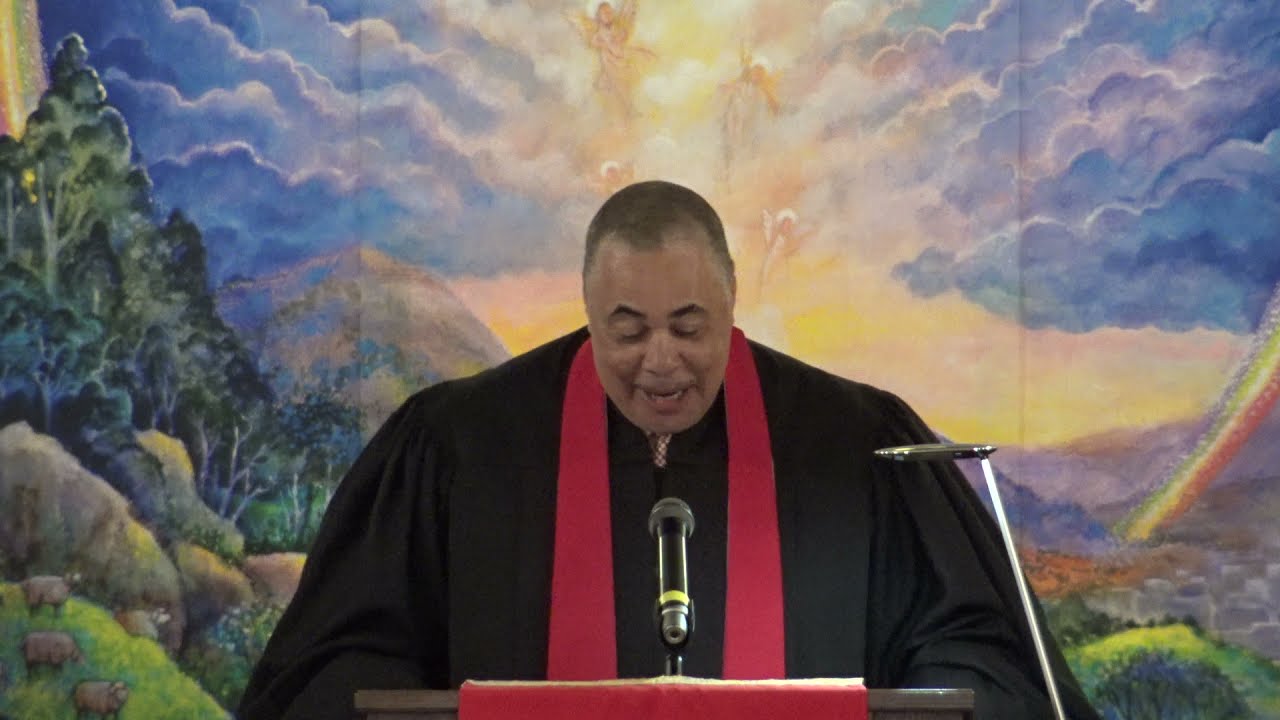This photograph captures a pastor or reverend, a large, dark-skinned man who might be Cuban or African-American, standing at a podium and delivering a sermon. He is dressed in a black priest robe with a red scarf draped around his neck. His short, slightly graying hair contrasts his dark complexion. The podium he stands at is adorned with a red fabric, and positioned near a black microphone. The background features an intricate mural depicting a vibrant hillside with goats, green trees, bushes, and rocks. Above the landscape, the sky is filled with purple and blue clouds, a yellow sun, angels near the light, and a vivid rainbow appearing on the right side. There's also a light above the podium illuminating the papers from which he reads.